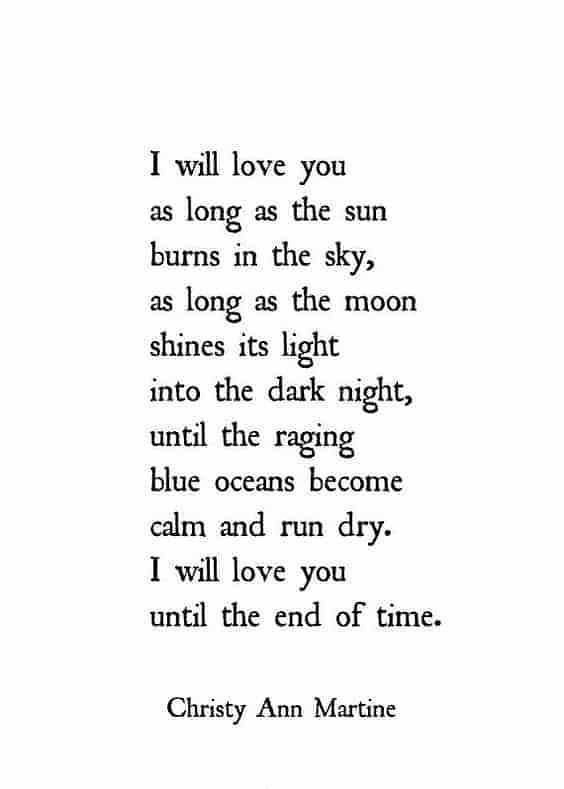The image features a white background with black text displaying a poem. The poem, 11 lines long and left-justified with all the left-most letters aligned, reads: "I will love you as long as the sun burns in the sky, as long as the moon shines its light into the dark night, until the raging blue oceans become calm and run dry. I will love you until the end of time." Below the poem, in smaller, centered print, is the poet's name: "Christy Ann Martine."